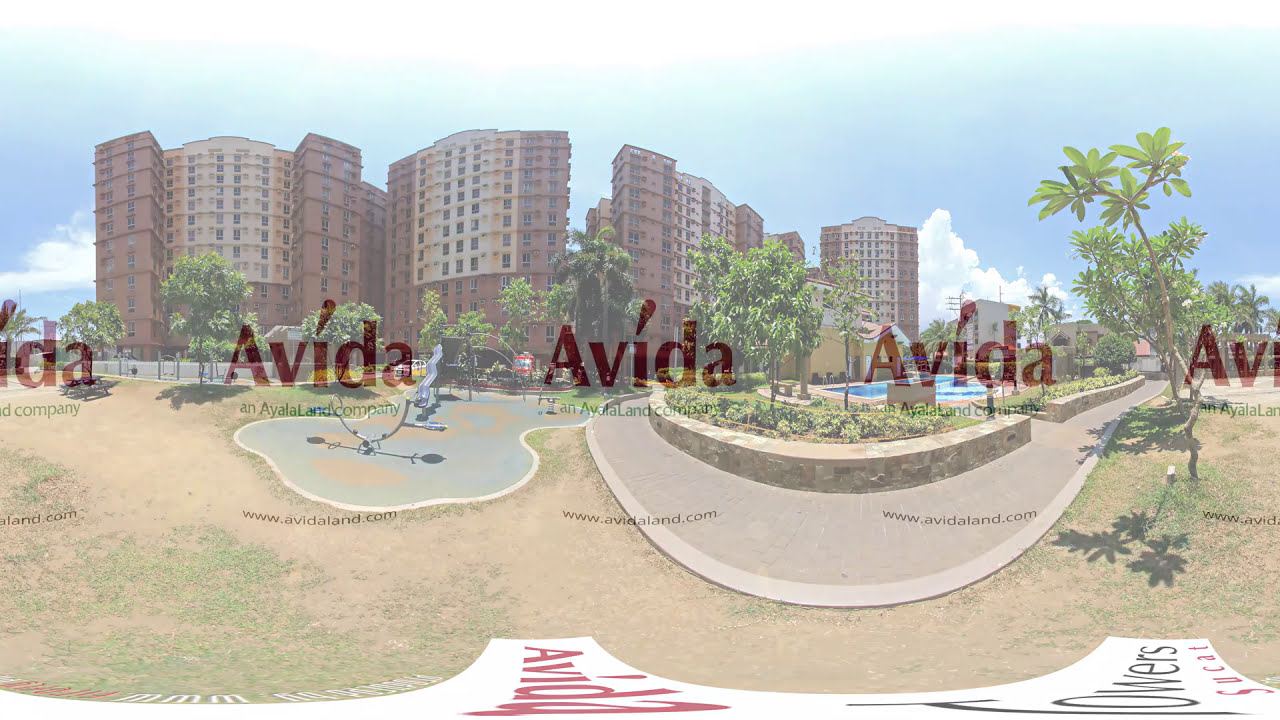The distorted lens effect in this panoramic image bends the straight lines slightly towards the viewer, adding a bowed-down appearance and a hazed overlay. Dominating the background, there are several multi-story buildings that appear to belong to a resort or a complex of condos, characterized by their uniform grid of windows and varying shades of reddish-brown to tan. Central to the image, the buildings are framed by lush green palm trees, contrasting with the clear blue sky scattered with white clouds.

In the foreground, a network of walkways curves towards the viewer, surrounded by patches of dirt and sparse grass. On one side of the path, a built-up section features decorative plants and bushes. To the right, there is a blue swimming pool, enclosed by a fence. A barely discernible sign sits in the lower-right corner, overshadowed by the repeated branding "AVIDA" in transparent dark red across the image. The scene captures a meticulous layout of an inviting resort environment with emphasized architectural uniformity and vibrant natural elements.